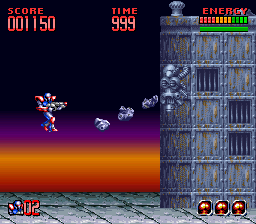This image is a screenshot from an early video game, likely from the Sega Genesis or Super Nintendo era, featuring detailed pixel graphics. Dominating the right half of the image, there's a formidable metal structure adorned with metal piles and a menacing face that appears to be shooting projectiles. The ground at the bottom of the image is a flat, gray stone surface. In the middle left, a character dressed in blue power armor with large red shoulder pads and wielding a small gun is seen floating. The user interface at the top of the image reveals, on the left, a red score reading "001150." In the center, a large "999" under the label "Time." On the right, the word "Energy" in red text with a long bar below it, split into thirds colored red, orange, and green. A small green rectangle is just below this bar. Additionally, in the bottom left corner, there's the text "O2," possibly indicating lives. The varying hues of the background transition from red and orange near the bottom to black at the top.